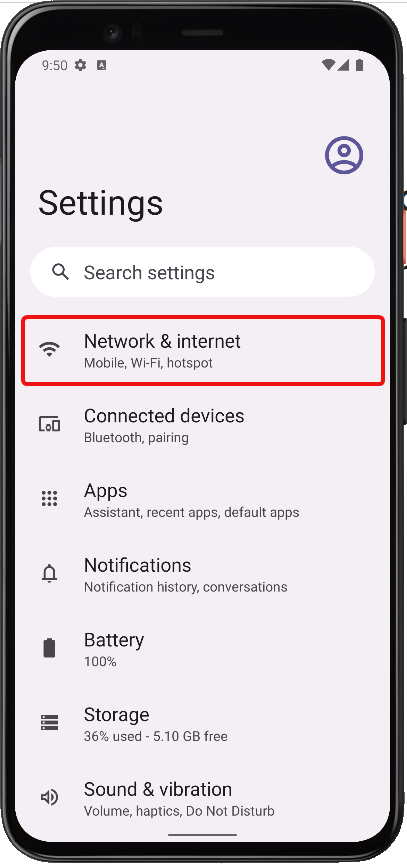The vertically oriented image shows a smartphone with a black rim resting on a white computer screen background. The black rimming of the smartphone is clearly visible, with some side buttons somewhat protruding. The upper part of the smartphone screen displays the time "9:50," followed by various icons on the top-status bar: a settings icon, a box with the letter "A," a Wi-Fi symbol, a triangle, and a battery life indicator.

Beneath this, there is a circular profile picture placeholder, alongside settings and a search bar that contains a magnifying glass icon and the words "Search settings." The main portion of the screen, set against a grey background, displays a list of settings menu options. These include: 

1. **Network and Internet** - Mobile, Wi-Fi, hotspot (highlighted with a red box).
2. **Connected Devices** - Bluetooth pairing.
3. **Apps** - Assistant, recent apps, and default apps.
4. **Notifications** - Notification history and conversations.
5. **Battery** - 100% charged.
6. **Storage** - 36% used, with 5.10 GB free.
7. **Sound and Vibration** - Volume, haptics, and do not disturb settings.

The detailed menu listing offers a glimpse into the various configurable aspects of the smartphone.